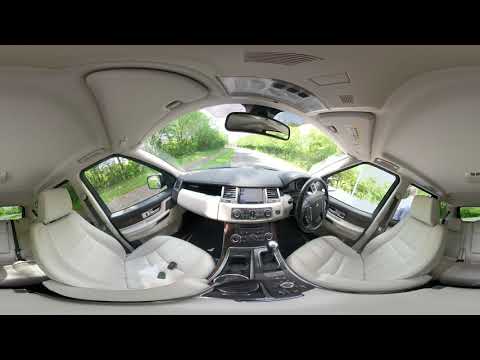This panoramic image of the inside of a newer model SUV or car, captured with a fisheye lens for a unique, distorted effect, reveals extensive details of its white and gray interior. The vantage point from the roof center emphasizes the front seats splayed apart, almost facing each other, with the driver’s side and steering wheel located on the right. The white fabric seats complement the white dashboard adorned with black accents and trim. Key features like the gear shift, GPS screen, radio console, rear-view mirror, side mirrors, and sun visors (currently up) are visible. Outside the vehicle, through the windshield and windows, a sunny day illuminates a gray asphalt road bordered by green trees and under a clear blue sky.